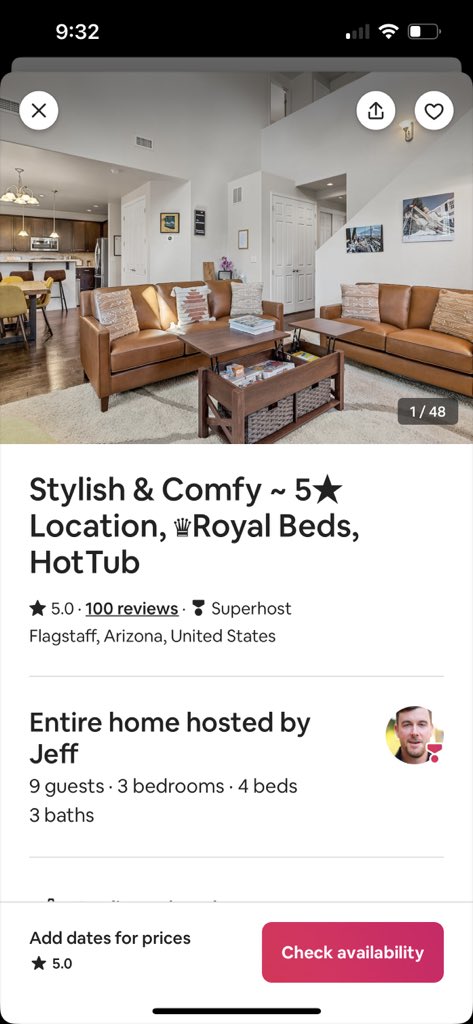This screenshot from a smartphone showcases a detailed listing for a rental home. The top navigation bar features the time "9:32" in white letters on the left, accompanied by icons for battery, Wi-Fi, and cellular service (one bar) on the right, all set against a black background. 

Below the navigation bar, there is an advertisement followed by the primary photo of the listing. The photo depicts a stylish living room furnished with a brown sofa and loveseat, a cream-colored rug, and framed pictures adorning the walls. The scene extends into a glimpse of the kitchen, featuring a chandelier above a dining table, additional wall pictures, and a staircase leading to an upper level.

The description beneath the photo reads: "Stylish and comfy, five-star location, Royal Beds, hot tub." Further down, it states the property has "5.0 stars from 100 reviews" and that the host is a "Superhost." The location is specified as Flagstaff, Arizona, United States, and the photo is labeled "1 of 48" in the lower right corner.

Additional details reveal that the entire home is hosted by Jeff and is suitable for nine guests, offering three bedrooms, four beds, and three baths. There is a prompt to "Add dates for prices," followed by a prominent red "Check Availability" button with white text.